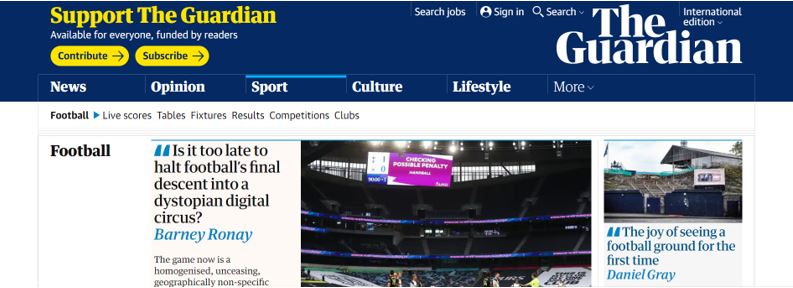The image appears to be a screenshot of The Guardian's website. The color scheme prominently features blue, yellow, black, and white. Headline text appears in blue, while calls to action such as "Support The Guardian," "Contribute," and "Subscribe" are highlighted in yellow. The Guardian's site title is displayed in white.

Central to the image is a main article with the headline: "Is it too late to halt football's final descent into a dystopian digital circus?" Next to it on the right, there's a smaller mini article titled: "The joy of seeing a football ground for the first time." Although they seem to share a thematic link, focusing on football, the content suggests they are separate articles. Above the articles, there's a navigation bar with search options, including "search sign" and "search jobs,” and The Guardian logo is positioned nearby.

The primary sections available for readers are listed at the top and include: "News," "Opinions," "Sport," "Culture," and "Lifestyle." The visible portion of the main article includes a picture of a stadium and mentions the author, Barney Ronay. The rest of the article content is not visible in the image.